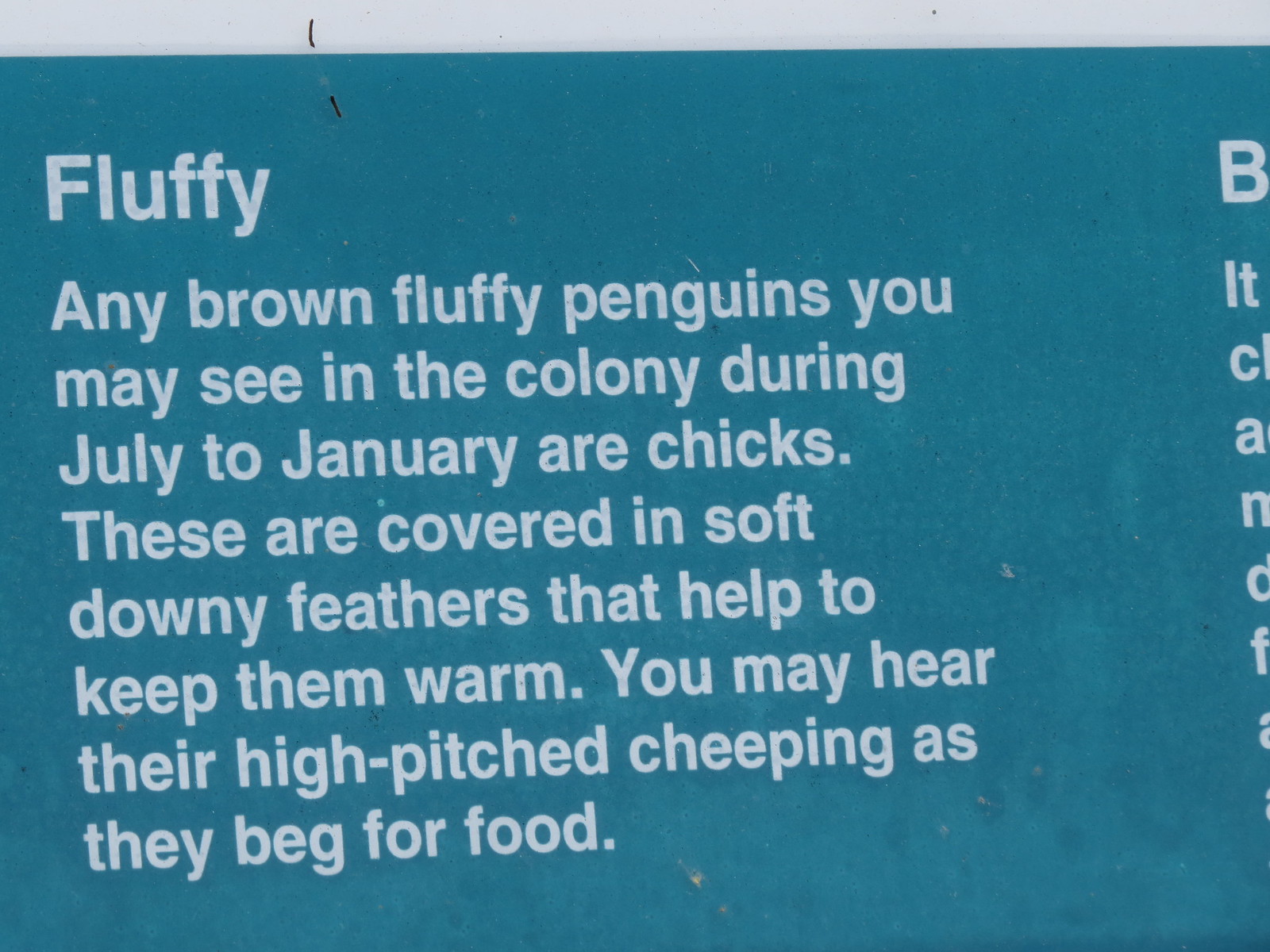This large square image captures a dark green information sign mounted on a white wall, likely at a zoo, detailing facts about penguin chicks. The sign's primary color is dark green, with a narrow white stripe at the top suggesting an outdoor, weathered material. In bold white letters at the top left, the heading "Fluffy" introduces the information. The text reads: "Any brown fluffy penguins you may see in the colony during July to January are chicks. These are covered in soft downy feathers that help to keep them warm. You may hear their high-pitched cheeping as they beg for food." On the far right side, another section begins with the letter "B", but only the initial letters of subsequent lines—'It', 'C', 'A', 'N', 'D', and 'F'—are visible as this portion is cut off by the image's edge. Additionally, there's a small black-and-white mark near the upper left of the sign, close to the 'Y' in "Fluffy," which could be a scratch or an additional mark on the sign.